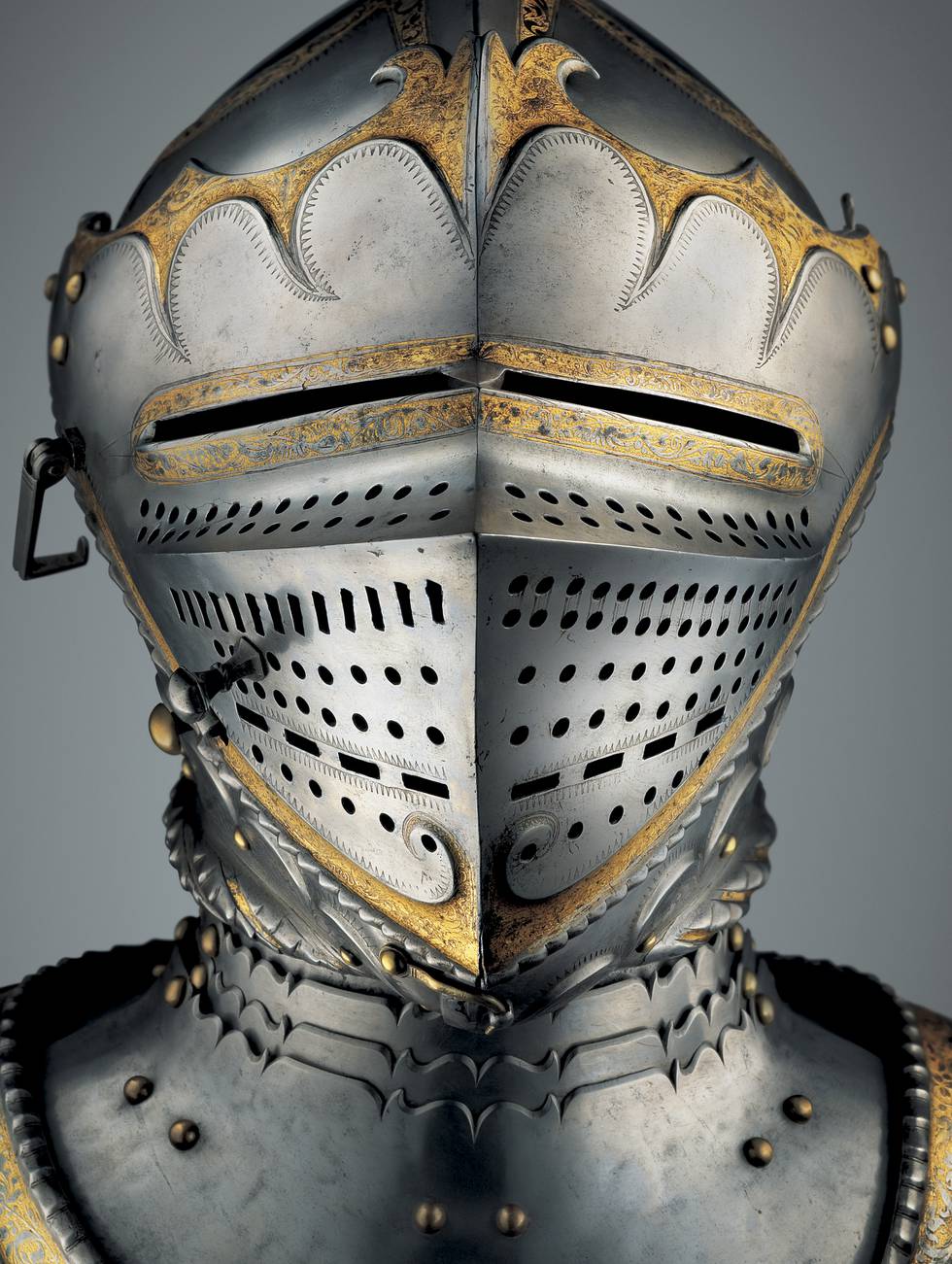The image captures an up-close photograph of a highly ornate helmet from a suit of medieval-style armor, displayed against a gray background. The helmet, crafted from dark-colored metal, features intricate gold trim that embellishes the crown-like headpiece. Gold accents surround the eye slits and span from the sides to the chin area of the helmet. Numerous holes of varying sizes are present on the front, around the nose, mouth, and cheeks. The neck armor appears substantial and includes triple layers secured with rivets, as well as a collar that also showcases rivets and gold embellishments. A latch is visible, attaching the face mask to the helmet, further enhancing the detailed craftsmanship of the piece.